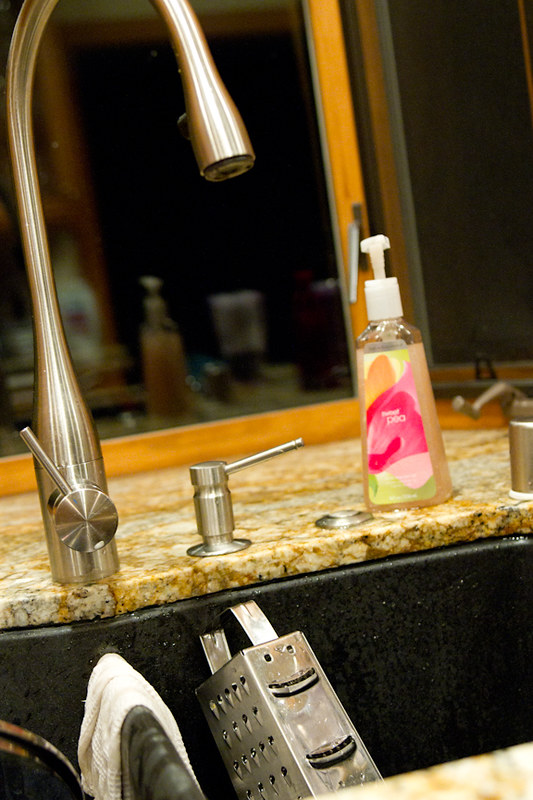This detailed indoor photograph captures a portion of a sink area, presented in portrait format and showcasing a mix of textures and elements. The countertop, featuring a striking black, brown, and white granite style, supports a sleek chrome faucet that elegantly curves up and down into the sink. Adjacent to the faucet is a matching chrome soap dispenser, seamlessly integrated into the sink. 

To the right of the soap dispenser sits a colorful bottle of liquid soap, with a vibrant label adorned in hues of orange, yellow, pink, and red, and marked with the text "Sweet Pea." The bottle is topped with a white pump handle, adding a touch of brightness to the scene. The black sink below them holds a metal cheese grater, which is leaning against its back wall, while a white cloth draped across the sink's divider adds a soft and practical element to the composition.

In the background, a wooden window frame can be seen, featuring a brown metal crank handle on the right. The window is dark, reflecting the items on the sink and contributing to the cozy, detailed atmosphere of the indoor setting.